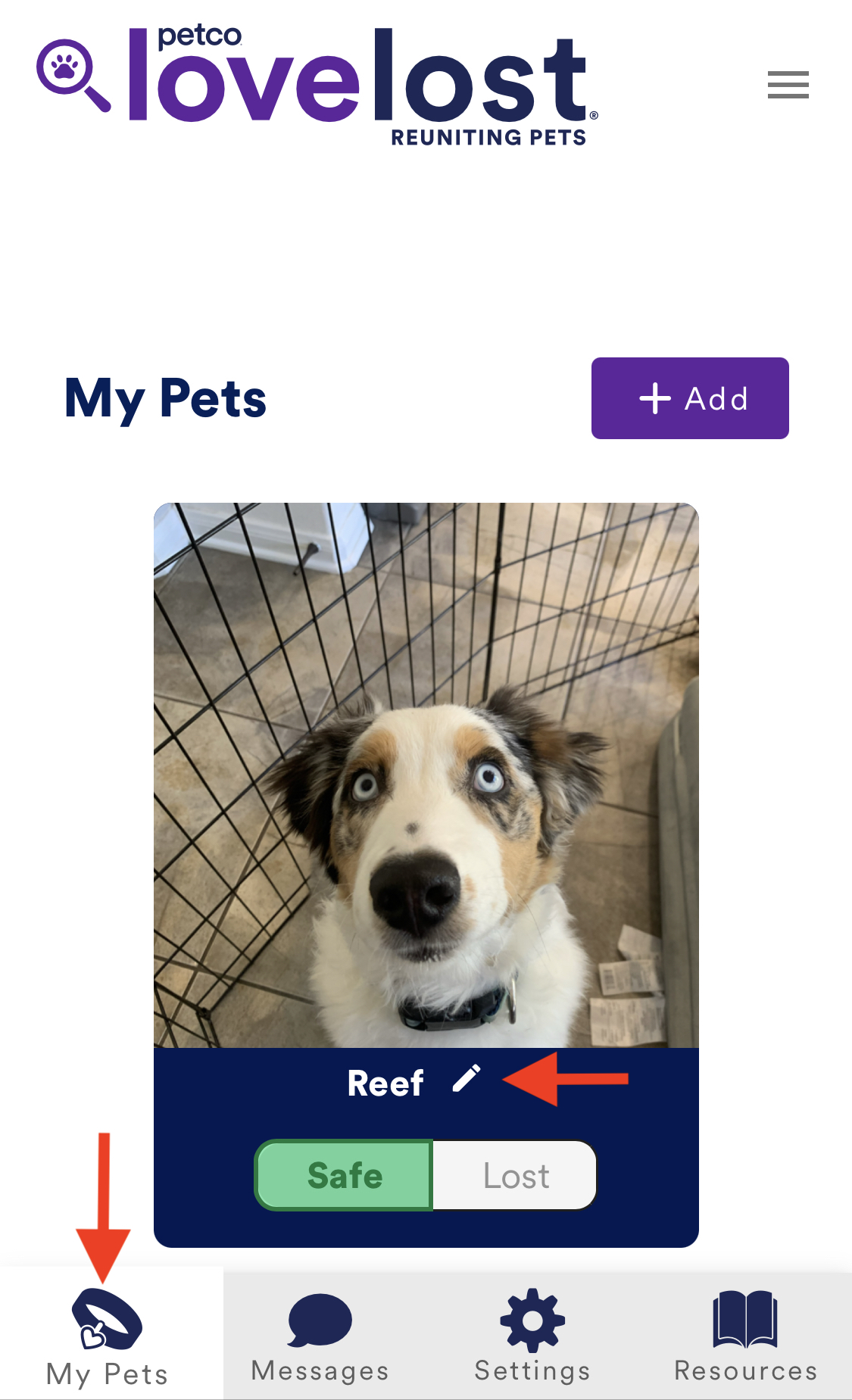The image depicts a furry dog with bright blue or white eyes and small pupils, staring directly into the camera. The dog is situated on a tile floor and enclosed within a black cage. The photograph is part of a website interface for "Petco Love Lost Reunited Pets," identifiable by its logo where "love" is in bright blue and "lost" along with the title appears in dark blue. A magnifying glass icon with a dog paw is located at the top left of the logo, and to the right, three horizontal bars are visible, suggesting a menu for additional options. Below the logo, there are icons labeled "My Pet" and a button marked with a plus sign for adding a pet. The dog's name, Reef, is displayed with two status options: "safe" and "lost," accompanied by an arrow pointing to a pencil icon next to Reef's name. Another arrow points to the "My Pets" section, which is adjacent to messaging, settings, and resource options.